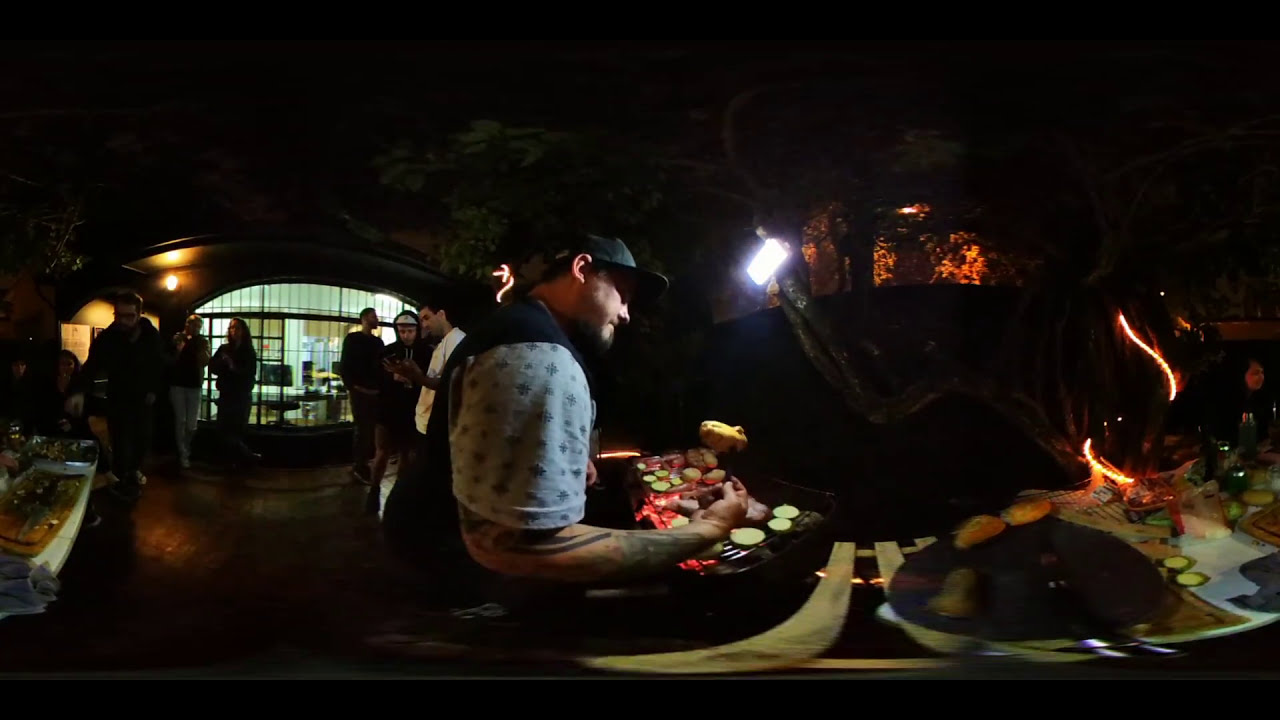In this nighttime indoor photograph, taken with a wide-angle lens that distorts and curves the surroundings, a man is grilling food in the center of what resembles a restaurant. The focal point is a white man wearing a gray short-sleeved shirt with gray markings and a baseball cap. He is extending his hand over a grill laden with pieces of vegetables and meat, possibly including potatoes and zucchini. An orange glow from squiggly lights or flames is noticeable to the right. 

The background is dim, with a notable arched window featuring multiple panes and framed by metal gates; beyond that, brightly lit areas suggest an office or store-like interior. The scene includes several other figures: a man in a white sash, another white man in a hoodie over a white baseball cap, and the silhouettes of a standing man and woman. Dark as it is, the image is illuminated by a small lamp hanging from the left side, shedding light on a nearby table set with various hors d'oeuvres. 

Additionally, a screen in the top right corner displays more orange flames, enhancing the warmth of the grilling scene. There is no text in the image, which captures a rich yet distorted array of indoor barbecue activity amidst a dark, bustling backdrop.